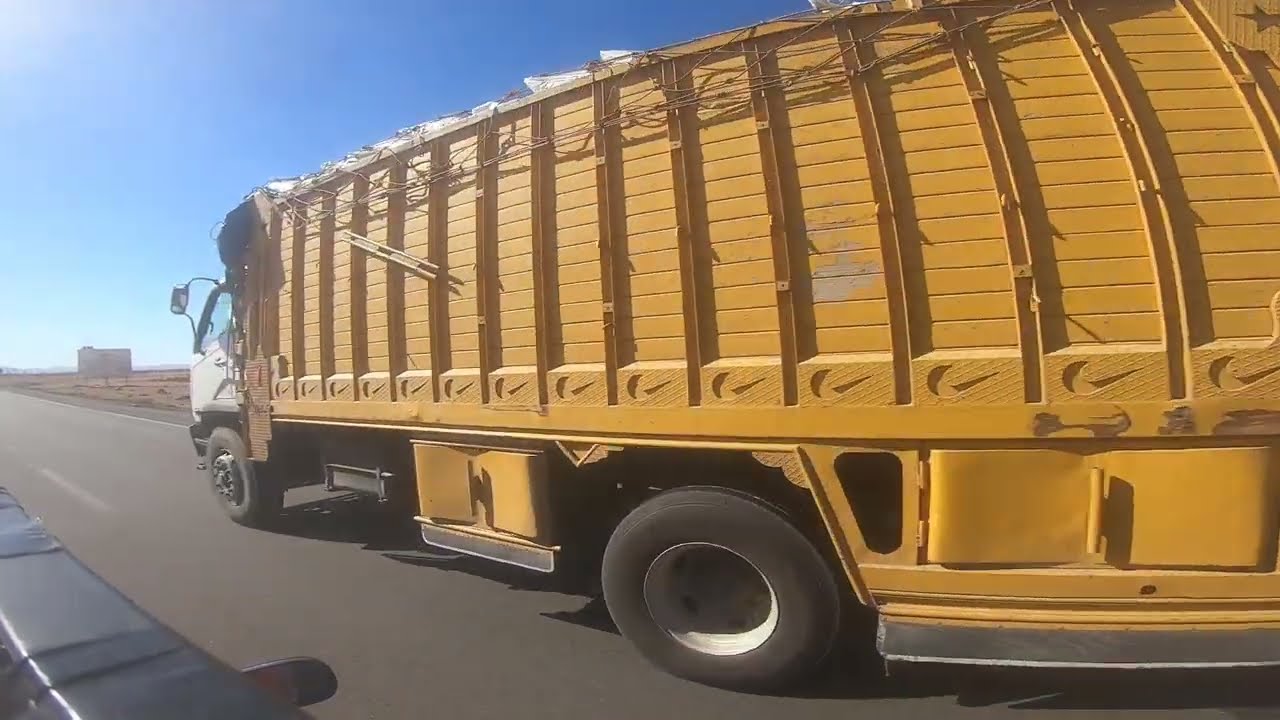This horizontally aligned rectangular image captures a yellow truck with a white cab occupying much of the frame, as it travels forward on a two-lane highway. The truck's wheels are black with white rims, and there are various pieces of wiring and cabling hanging down the side. The sky above is a light blue with very few clouds, providing a clear, bright backdrop. The road is light gray asphalt, marked with a dotted white line indicating lanes. To the right of the road stretches a largely flat, desert-like landscape in shades of brown and dark brown. In the distance, on the right side of the road, a blurry rectangular building is visible. Additionally, there is a partial view of another vehicle to the left of the truck, with only a side mirror and part of its side visible. There's also a white road sign with black lettering on the side of the road. Overall, the scene depicts a truck driving through a sparse, possibly hot environment, heading towards its destination.